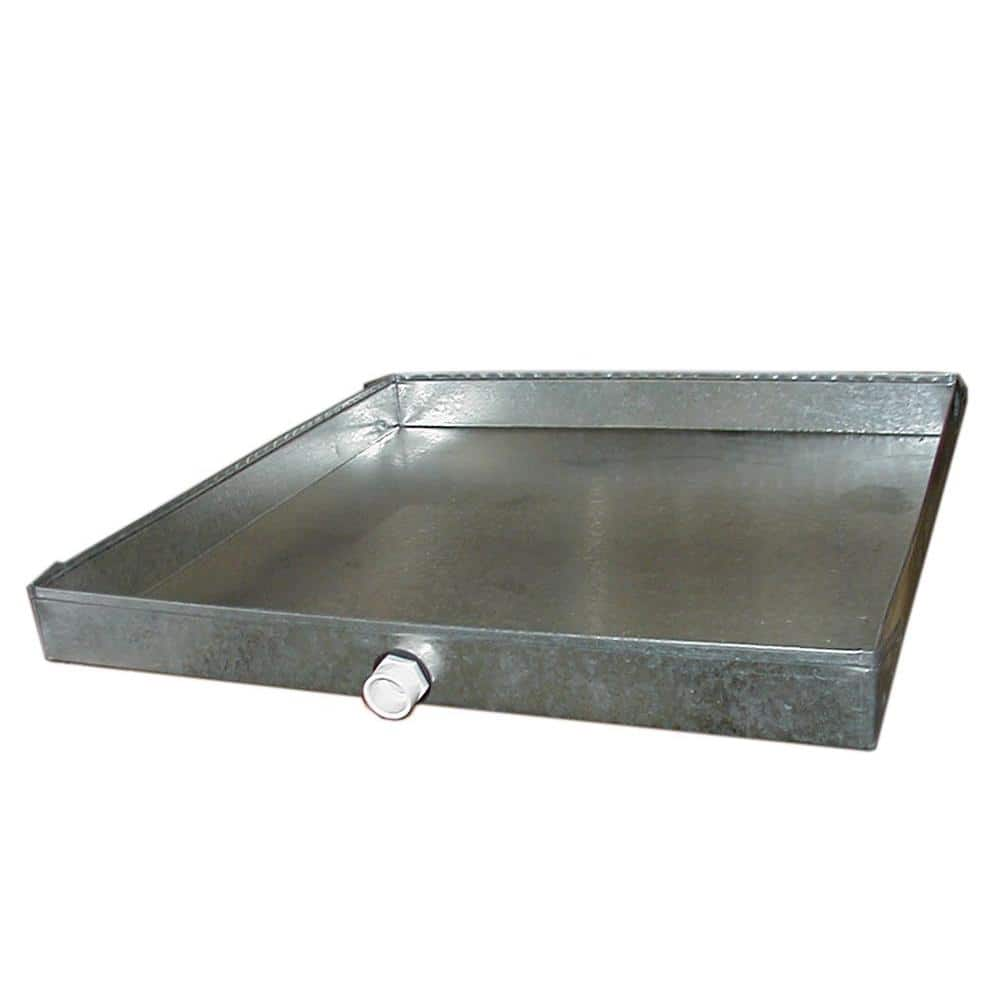This highly detailed photograph or extremely realistic drawing showcases a sturdy, silver metal pan, likely part of a professional kitchen setup. The pan is oriented diagonally to the left, emphasizing its rectangular shape that is wider than it is long, with approximate dimensions of two feet in width, one and a half feet in length, and an inch and a half in height. The interior of the pan displays various shades of gray, suggesting a well-used surface; there's a prominent stain on the right and a reflective, shiny spot in the upper left. Attached to the front side of the pan is a distinctive, white, hexagonally-based knob or nozzle with a circular top, indicating it may be an adjustable component. The background is pristine white, further highlighting the pan's utilitarian design and giving the entire image a clean, professional look.